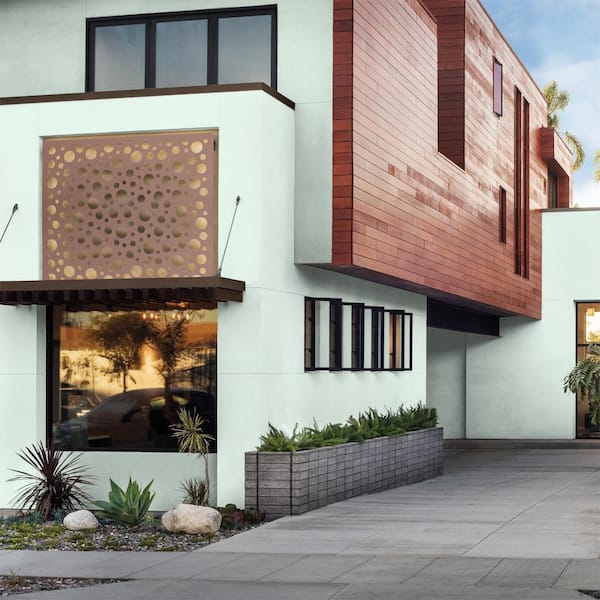The image captures a modern and minimalistic house, characterized by its rectangular design and clean lines. The front yard features a concrete paver driveway and a brick sidewalk adorned with desert plants, including aloe, on rocks and pebbles. To the left of the driveway, there is a large, modern house distinguished by its white stucco surfaces and contrasting reddish wooden panels covering the right side. The front façade showcases a blend of materials, including a section with golden and brownish-white accents resembling bubbles, and multiple open windows outlined in black frames. A notable planter box with green plants is situated next to the house, complementing the greenery along the front and side. The building also has a second floor with a wall that juts out, decorated with wood strips and various indentations, adding to the modern aesthetic. The scene is set on a sunny day with a bright blue sky and scattered white clouds, enhancing the modern vibe through the reflections on the windows and the overall landscaping.